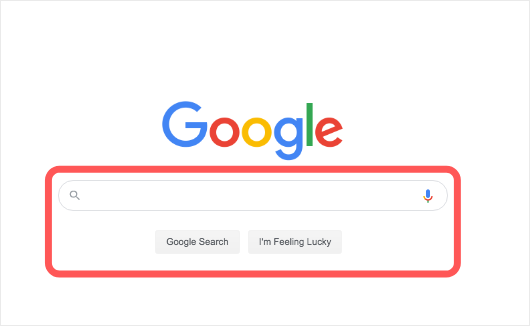The image displays a screenshot of the Google homepage. The page is enclosed in a thin, gray rectangular border, with a white background filling the inside. At the top of the page, there is some empty white space. Centrally located on the page is the Google logo, featuring a capital "G" in blue, a red "O", a yellow "O", a lowercase "g" in blue, a green "l", and a lowercase "e" in red.

Beneath the logo is an oval-shaped search bar with a light gray outline. On the left side of this search bar, there is a gray magnifying glass icon, indicating the area where users can type their search queries. To the right of the magnifying glass is a microphone icon with a blue head and a red body, supported by a green stick, allowing users to input search queries via voice.

Below the search bar, there are two horizontally aligned rectangles with light gray outlines. The left rectangle contains the text "Google Search" in black, while the right rectangle displays the text "I'm Feeling Lucky," also in black. The entire search engine interface, including these two buttons, is framed by a red border.